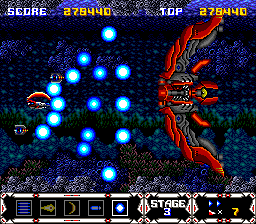The image depicts an older computer game reminiscent of the 1990s, characterized by its classic pixelated graphics. At the top of the screen, a score of 270,440 is prominently displayed, matching the top score. The game is a side-scrolling shooter where a player-controlled ship is actively firing bullets at a formidable red and black creature. 

The bottom portion of the screen features a control panel with various weapon options that players can toggle through. The currently selected weapon is represented by orbs. Other available weapons include four straight lines indicating a multi-directional shooter, a bolt-like shape, a curved line resembling a parenthesis, and a straight line with a dot at the end which suggests a standard bullet. 

Additionally, the status bar indicates that the player is on Stage 3. Adjacent to this stage information, there is a small icon accompanied by the text "time 7," providing further gameplay details.